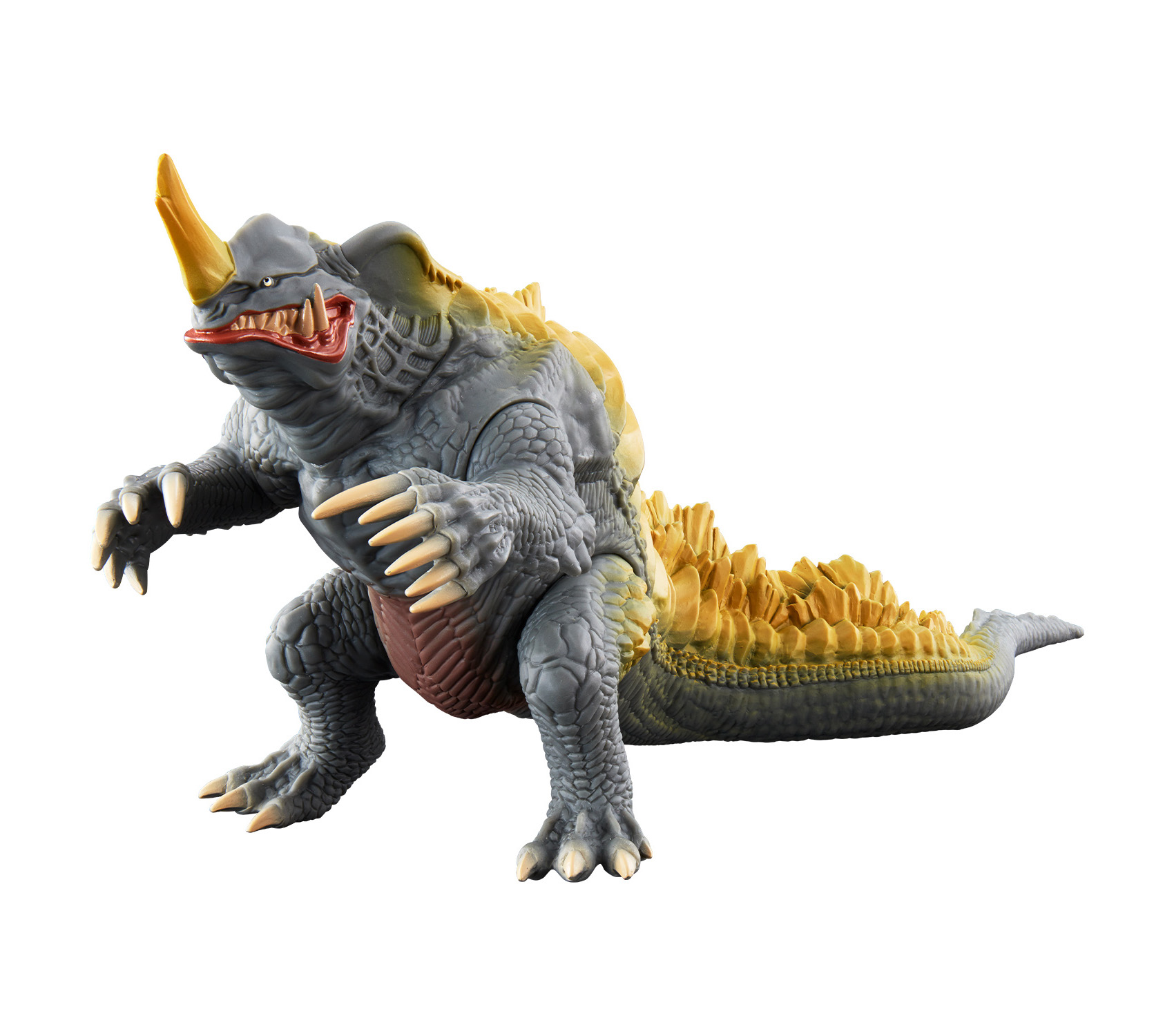This image depicts a highly detailed fantasy-style reptile monster, which appears to be a toy or figurine, possibly made from plastic or resin. The creature is crouching menacingly, its powerful, lizard-like body primarily gray with a brick-red underbelly. It has a long tail adorned with several rows of yellow, tooth-like ridges that extend up its back. The monster's hands are large, with six long, sharp talons on each hand, while its feet have three toes. Its face is articulated with tiny eyes, a very large gold horn protruding from its forehead, and a mouth filled with large, protruding teeth. The monster’s overall appearance, complete with webbed legs and what seems to be a protective breastplate, suggests a formidable and intimidating fantasy creature.